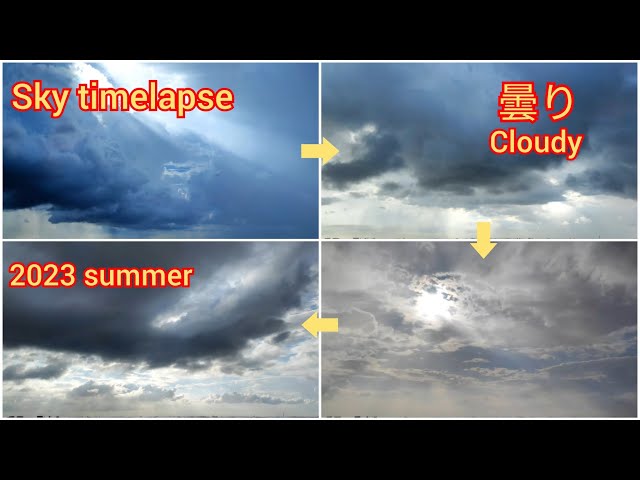This image is a landscape-oriented collage consisting of four rectangular panels, each depicting a section of a clouded sky. The collage is bordered thickly with black bars on both the top and bottom. Yellow arrows connect the panels in a clockwise direction, starting from the upper left to the upper right, then to the lower right, and finally to the lower left.

In the upper left panel, dark blue thunderclouds tapering to lighter shades are accompanied by the text "Sky Time Lapse" in beige with a reddish-orange outline. The upper right panel, also featuring dark clouds with a lighter sky at the bottom, bears the word "Cloudy" in yellow, alongside some Japanese or Thai characters. The lower right panel mirrors the sky theme without any textual labeling. Finally, the lower left panel displays the text "2023 Summer" in yellow letters. All panels show mid- to high-level clouds that are predominantly bluish-gray. The overall design gives a sequential and thematic representation of the sky across different times or conditions.